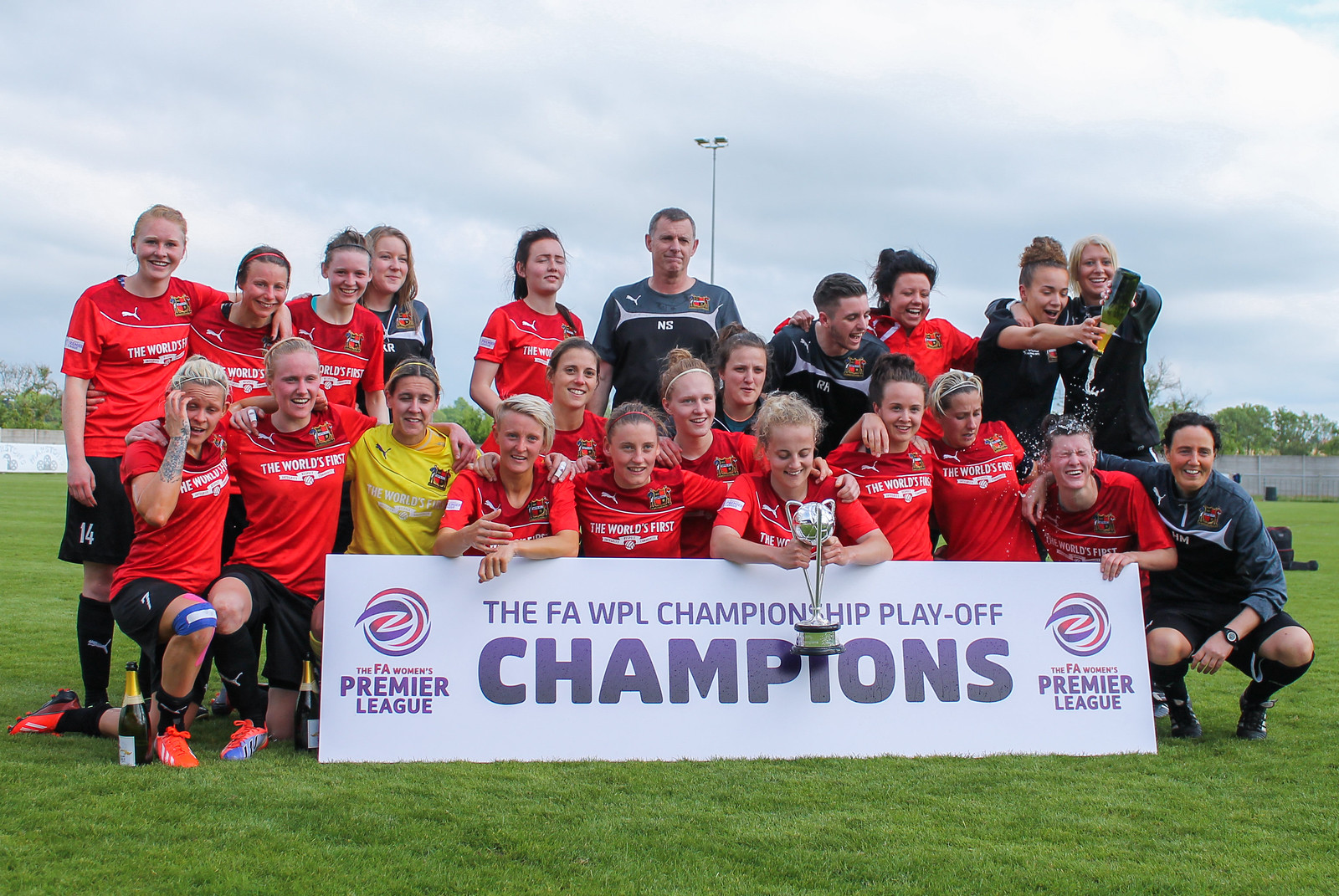The photograph captures an all-female soccer team celebrating their victory in the FA Women's Premier League Championship Playoff, posing joyfully on a lush, green soccer field. The team is arranged in three rows, with a mix of standing, sitting, and kneeling players, all clustered around a placard that reads "FAWPL Championship Playoff Champions." Most of the players are wearing red jerseys, while one, presumably the goalie, is sporting a yellow jersey. The head coach, wearing a black jersey, stands in the middle of the back row. Another man, likely part of the coaching staff, is celebrating beside him in a gray and black t-shirt. A particularly jubilant moment is captured as one team member on the right side pours a bottle of champagne over another's head. The atmosphere is electric with happiness, as the predominantly Anglo-Saxon, Caucasian young women smile broadly, united in their shared triumph under a cloudy sky.